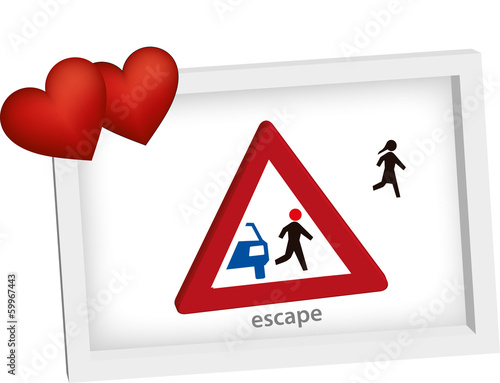This digitally-created stock image features a central, bright red triangle displayed on a light gray rectangular background. Within the triangle, a stylized depiction of the right portion of a blue vehicle can be seen. Adjacent to this vehicle, there's a simple illustration of a person with a red circle for a head, appearing to walk or run away from the vehicle. This triangle is framed in white. Below the triangle, the word "escape" is written in lowercase letters.

In the upper left corner of the image, there are two shaded red hearts, adding a whimsical touch. Meanwhile, in the upper right corner, another stylized figure in black is shown walking away from the triangle’s edge. All elements, including the images and text, are subtly positioned at a diagonal angle, contributing to the dynamic feel of the artwork. The overall color scheme features white, gray, red, blue, and black, with a note that the image bears the watermark “Adobe Stock.”